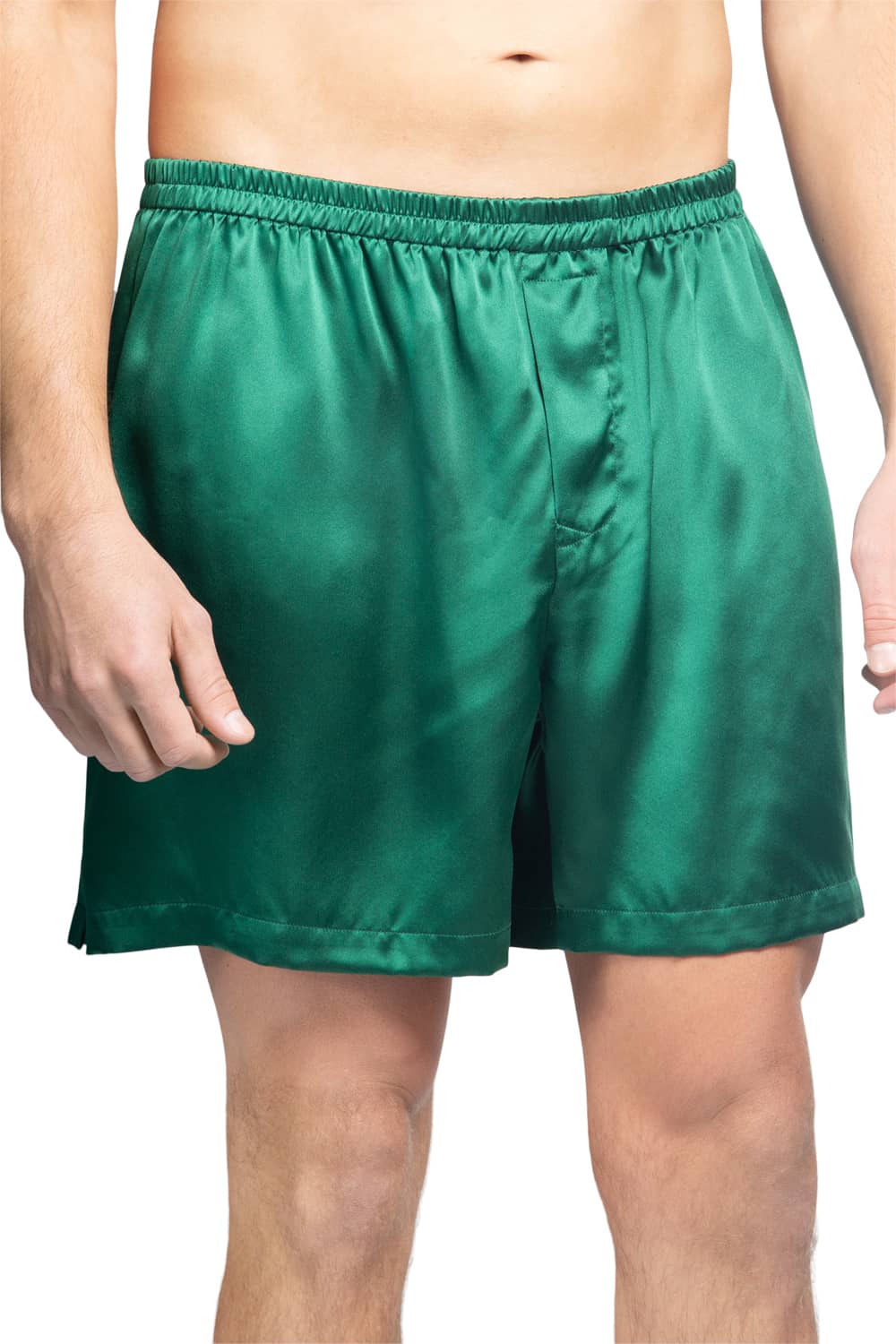The image features a close-up of a fashion model wearing bright green, shimmering boxer shorts made of a silky or satin material. The boxer shorts have an elastic waistband and a sewn hem at the bottom of each leg, giving them a loose, crinkled appearance. The model, a thin, pasty Caucasian male, is depicted from his belly button to just below his knees. He is shirtless, revealing his bare legs and body hair, but his belly is hairless. His arms are positioned at his sides, a few inches away from his body. The photograph is set against a plain white background and appears to be an advertisement, likely for a clothing catalog or website. The model looks relaxed and is showcasing the boxer shorts effectively, with no other distracting elements in the shot.